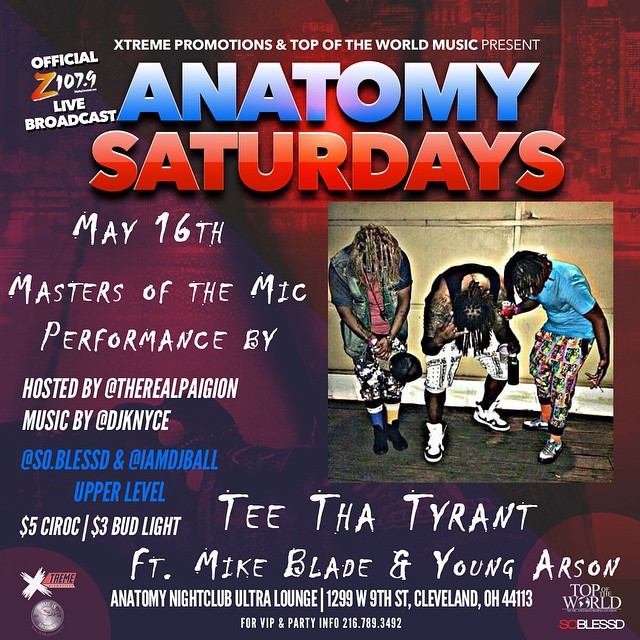This is a vibrant and detailed advertisement poster for a music concert titled "Anatomy Saturdays," prominently promoted by Extreme Promotions and Top of the World Music, with an official live broadcast from the radio station Z107.9. The background displays a mix of red and black hues featuring abstract artwork, setting a dynamic stage. The title "Anatomy Saturdays" stands out, with "Anatomy" in bold blue uppercase letters over "Saturdays" in striking red uppercase letters. Above the title, in smaller white all-caps text, it reads "Extreme Promotions and Top of the World Music Present." The left side of the poster details event specifics: "May 16th Masters of the Mic Performance by" followed by the hosts and performers, with mentions of @TheRealPagan and DJK NYCE, along with mentions of additional acts @So.Blessed and @IMMJD Ball. The poster highlights drink specials, such as $5 Ciroc and $3 Bud Light. Centered at the bottom, it announces performances by T Tha Tyrant, Mike Blade, and Young Arson. The venue, Anatomy Nightclub Ultra Lounge, located at 1299 West 9th Street, Cleveland, Ohio 44113, is emphasized in white all-caps text. In the lower-right corner, the promotional credits are reiterated with "Top of the World" and "So Blessed." The poster also includes an image of three musicians in dynamic, bent-over poses, wearing brightly colored clothing, suggesting a lively and engaging atmosphere for the concert.